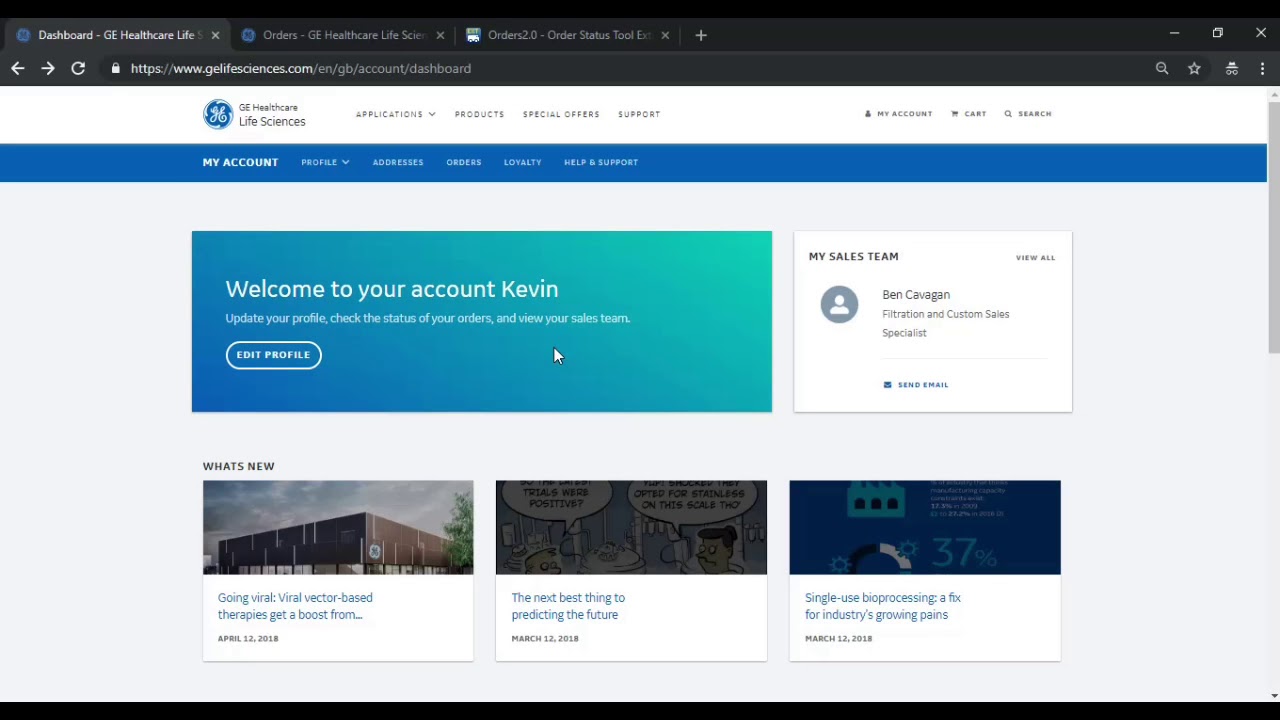In the upper section of the interface, the background is painted black. On the left side, there is a small blue circle, followed by the text "Dashboard - GE Healthcare Life." Below this, the search bar displays the URL www.gelifesciences.com/account/dashboard. 

Within this area, there is a blue circle enclosing the cursive white letters "GE," situated next to the text "GE Healthcare Life Sciences." Further to the right, navigation options are listed: "Applications," "Products," "Special Offers," and "Support."

Beneath this main header, a two-tone box is presented: the left half is blue and the right half is green. Inside, a welcome message reads: "Welcome to your account, Kevin. Update your profile, check the status of your orders, and view your sales team." Within a highlighted circle, there is an "Edit Profile" prompt.

To the right of this, in a white square labeled "My Sales Team," the text displays the name "Ben Coggin." 

Below this section, there are three different content squares under the heading "What's New." The first square features an image of a building. The second square has the text "The next best thing in predicting the future." The final square reads "Single-use bioprocessing: a fix for industry's growing pains."